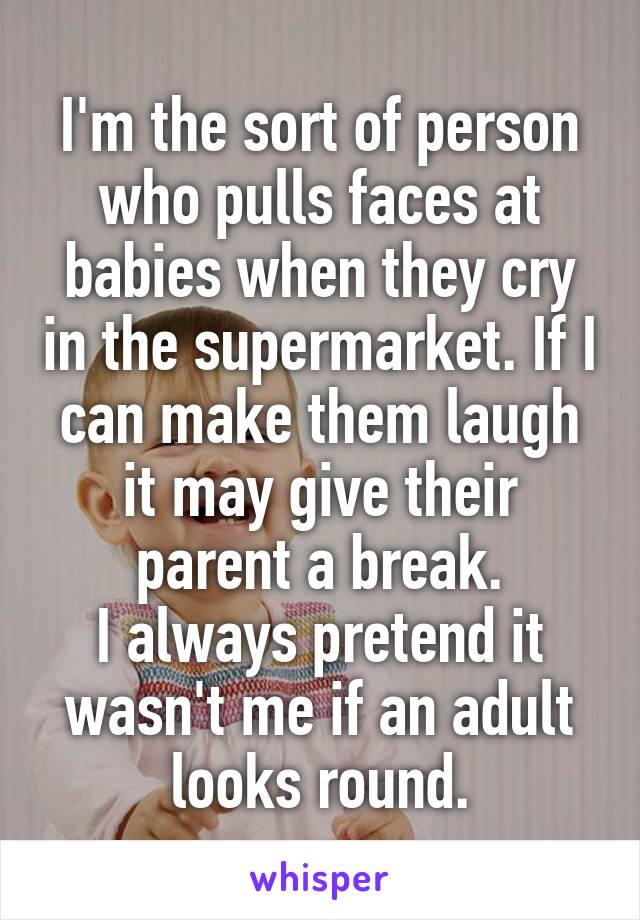A close-up image shows a baby with fair skin and blondish-brown hair, visibly crying with its eyes squinted or closed, mouth open revealing a couple of bottom teeth, and small fisted hands. The baby, wearing a white long-sleeved top with colorful horizontal stripes across the chest and shoulders, is positioned in the background to the middle to lower left portion of the image. The backdrop features a dull, grayish-brown rectangular shape with narrow vertical stripes that fade from darker at the top to lighter towards the bottom. Transposed over the entire image in white font is the text: "I'm the sort of person who pulls faces at babies when they cry in the supermarket. If I can make them laugh, it may give their parent a break. I always pretend it wasn't me if an adult looks around." The word "whisper" appears at the very bottom in lowercase blue letters against a strip of white background.